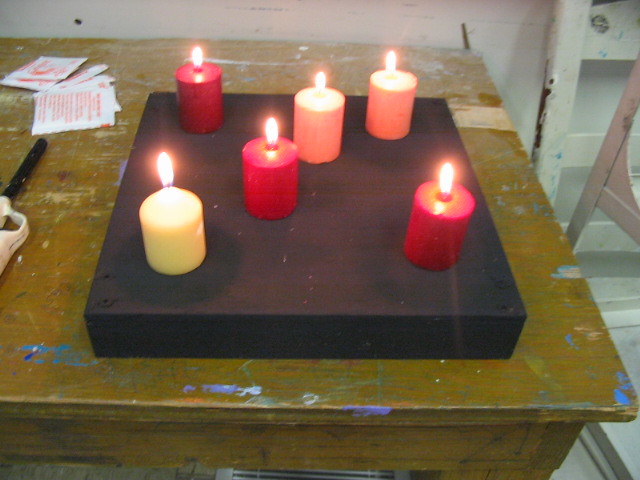The image depicts a well-used wooden tabletop, likely used for arts and crafts, with a multitude of paint splatters in various colors—predominantly blues and whites—along with visible scratch marks and debris. At the center of this chaotic yet creative space lies a black, square platform about an inch high. Arranged atop this platform are six lit votive candles in varying hues: a red one in the upper left, a yellow one in the lower left, two pink ones towards the upper right, and two more red ones, one positioned just down and left of center and the other in the lower right. Scattered around the table are additional craft-related items, including a white-handled lighter with an extended lighting part on the left and what appear to be small packets or teabags with orange text and symbols in the distance, particularly in the upper left. To the right of the image, parts of a metal stand and a painted metal object resembling a ladder can be seen, though they are mostly cut off from view. The entire scene exudes a sense of creative clutter, indicative of numerous art projects.